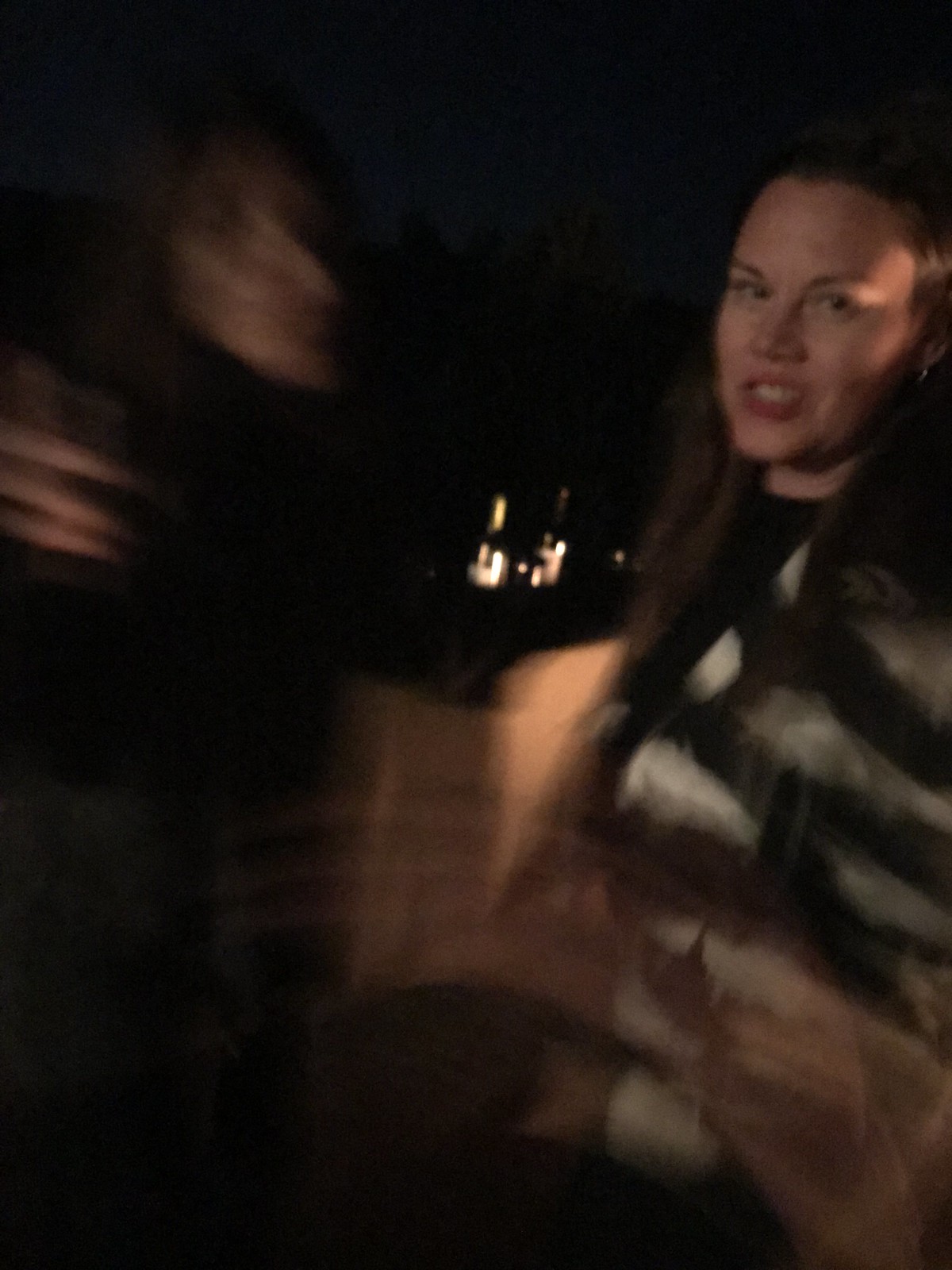This image captures a nighttime scene featuring two Caucasian women. The photograph has a double-exposed and blurry quality, creating an almost surreal effect. The woman on the right, who is more clearly visible, has long brown hair and is wearing a black and white striped jacket over a black undershirt. She is facing the camera but standing slightly to the side, and a light casts a glow on her temple. Her expression appears to be a scowl, and she seems to be holding an indeterminable object due to the picture's blurriness. The woman on the left is much harder to discern; her features are highly blurred and stretched, making it difficult to gather details about her appearance. The background reveals a dark cityscape with some lit-up buildings, contributing to the image's nighttime setting. There are also lights in the background between the two figures, adding some illuminated glows to the otherwise dark scene.